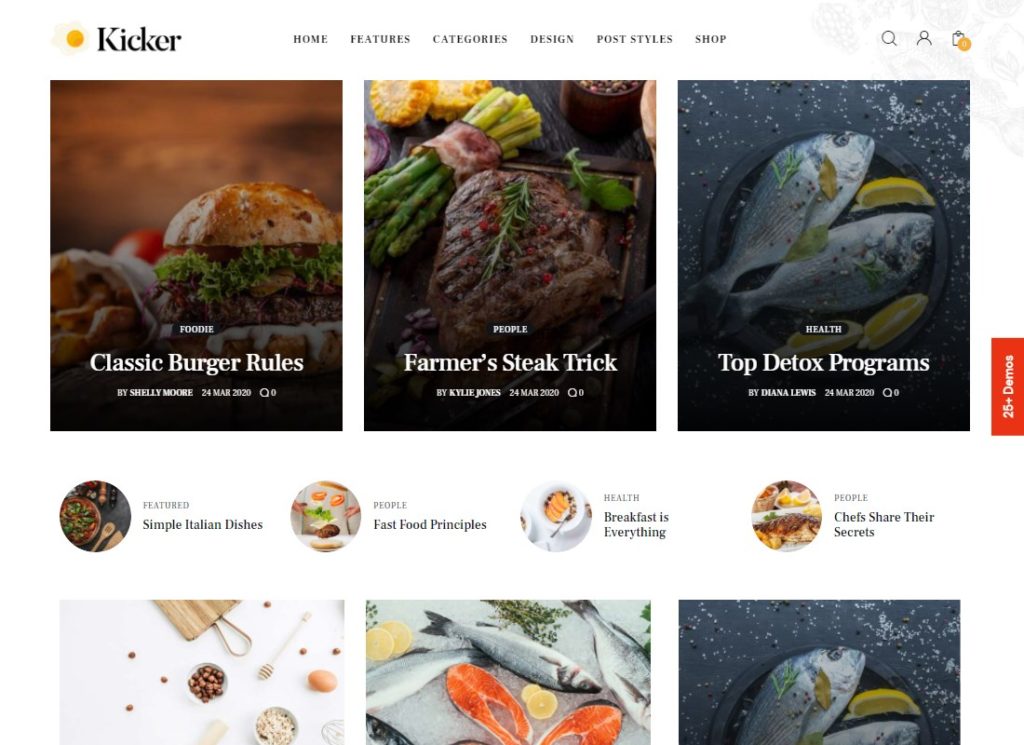Here is a cleaned up and detailed descriptive caption for the image:

---

This image depicts the homepage of a website called Kickr, set against a white background. Prominently displayed at the top is the website's name "Kickr" in bold black letters, accompanied by a distinctive logo featuring an open egg yolk.

To the right of the logo, the navigation bar includes links for Home, Features, Categories, Design, Postals, and Shop. Adjacent to these links are three icons: a magnifying glass for search, a person icon likely indicating user account options, and a clipboard icon with a yellow notification badge, suggesting alerts or updates.

Beneath the navigation bar, there is a row of featured food articles. The first article, titled "Classic Burger Rules," is authored by Shelly Moore and dated March 24, 2020. It features a speech bubble icon indicating zero comments and a background image of a small burger stacked with lettuce.

The second article, "Farmer's Steak Tricks," by Kylie Jones, also dated March 24, 2020, and showing zero comments, includes an enticing image of a steak garnished with vegetables, accompanied by celery, and presented on a fancy tray.

The third article, "Top Detox Programs" by Diana Lewis, dated March 24, 2020, tagged under "Health," depicts two silver fish on a black plate, sprinkled with what appears to be salt.

Following this row, a section marked "Featured" displays three more articles. "Simple Italian Dishes" features an image of an Italian dish. "Fast Food Principles," tagged under "People," shows an image within a circle of two hands tossing food. "Breakfast is Everything," tagged under "Health," depicts a cereal with orange slices and a spoon.

Lastly, the article titled "Chefs Share Their Secrets," tagged under "People," features an image of grilled fish.

At the bottom, three partially visible images display a variety of nuts and grains in white bowls on a white table with a cutting board and honey stick, a prepared salmon dish with cut-open pieces, lemons, and vegetables, and a repeat of the "Top Detox Programs" image.

---

This detailed caption provides a comprehensive, structured overview of the website’s layout, highlighted features, and content, capturing the visual essence of the Kickr homepage.